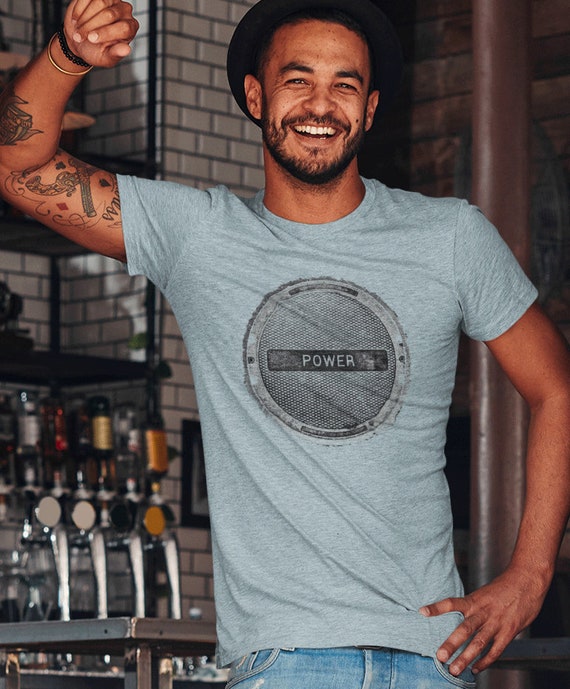The image depicts a man standing and smiling warmly, appearing to be in a bar or restaurant. He has a tanned, light African American complexion and brown eyes. He sports a bit of facial hair including some scruff and a partial beard. His brown eyes are set under the brim of a black fedora-style hat. His attire includes a gray T-shirt with the word "POWER" emblazoned in the center, within a black strip and circle design, paired with blue jeans, the tops of which are just visible. His left hand rests on his hip, while his right arm is raised, possibly resting on a shelf, showcasing tattoos on his forearms. He wears a black bracelet and a gold bangle on his right wrist. The background features white subway tiles and beverage taps, alongside a brownish-red support post and some ironwork, enhancing the ambiance suggestive of an industrial-style bar setting.